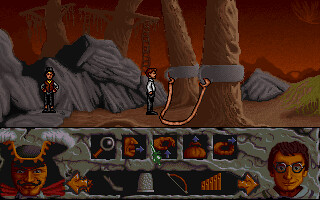This is a detailed color screenshot from a video game, showcasing both the environment and characters. The image is divided into two sections. At the top, against a backdrop of rocks and a striking red sky, stands a character with hands on hips, wearing a black top hat, glasses, a red vest, a long-sleeved white shirt, and black pants. In the center, a character is shown in profile, facing right; they have short red hair, a white long-sleeved shirt, and black pants. Two tree trunks, wrapped with wide metal bands and connected by a long rope, anchor the middle of the image.

The bottom section displays the inventory screen, featuring two distinctive cartoon figures. On the left is a menacing pirate, with a wicked smile, a cleft chin, and psycho eyes. He sports a black handlebar mustache with curled ends, dark black hair with red accents, and a black hat adorned with gold trim that curves upward. On the right, there is a character reminiscent of Bill Gates: a human with a yellow face, wire-rim glasses, brown hair, pale to dark beige skin, and a smirk. This bottom section also includes icons of weapons positioned between the two characters. The intricate details and style suggest an older video game, adding a nostalgic charm to the scene.